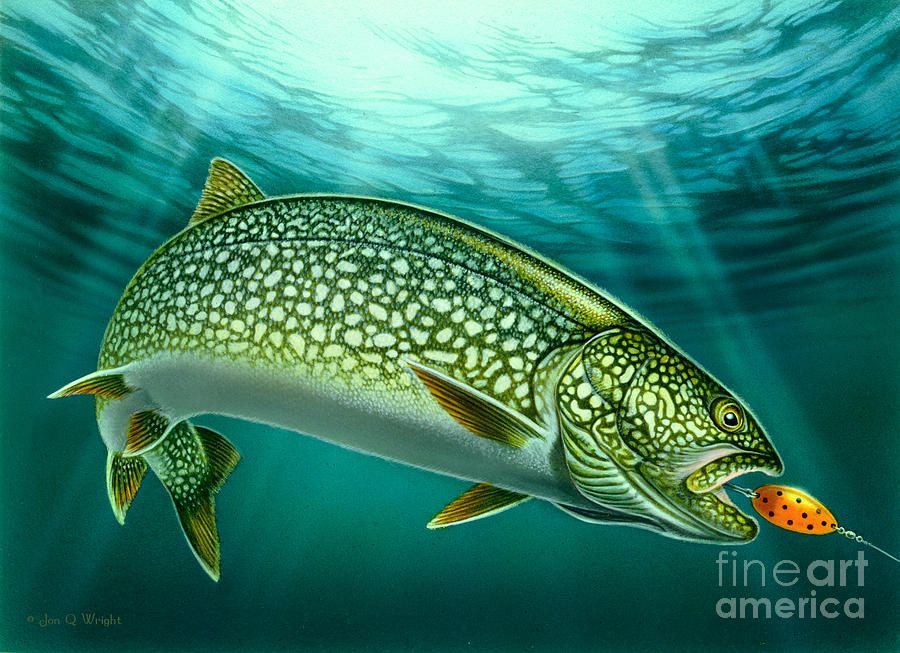This is an angled, rectangular, computer-generated graphic of a bass fish captured under the water, depicted about to bite an oval-shaped orange and black lure attached to a silver string and hook. The large fish, predominantly green with white spots and a fully white belly, features green fins tipped with orange and some yellow speckles across its body. The fish, mouth open toward the hook, is illuminated by rays of sunlight shining through the water above, creating a dynamic, underwater atmosphere. The image also includes a watermark reading "Fine Art America" in the lower right-hand corner and the name "John Q Wright" in the lower left-hand corner.